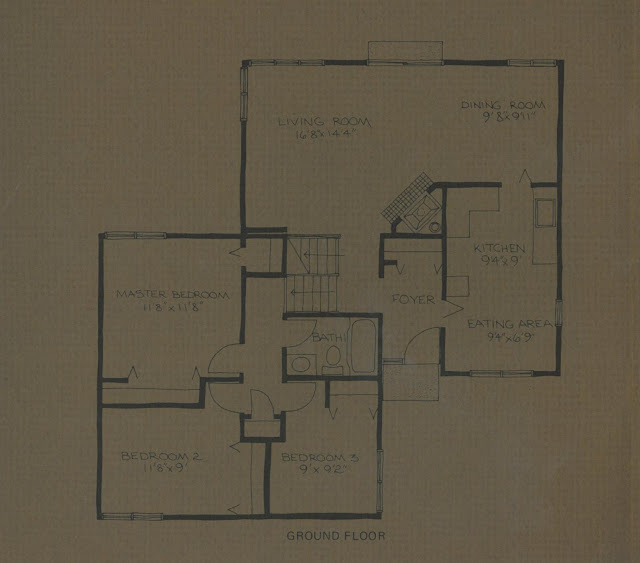This image depicts a detailed, pencil-sketched floor plan of a house, rendered on dark paper. The layout is organized into two overlapping squares: one located in the bottom left corner, extending into the top right corner.

On entering the house through the front door, there is a foyer. To the right of this foyer, a connected area incorporates an eating space and kitchen, which seamlessly flows into an adjacent dining room. To the left of the foyer lies a spacious living room. From the entrance, turning left leads to a stairwell that ascends to the second floor.

The upper floor, accessible via this stairwell, comprises a landing that opens up to several rooms. To the immediate right of the landing is the master bedroom. Straight ahead are two additional bedrooms, designated as bedrooms two and three, which are positioned next to each other. Situated next to these secondary bedrooms is a shared bathroom.

Accompanying these sketches are the precise dimensions of each room, demarcations of closet spaces, and the exact placement of the staircases. Such detailed plans are typically provided by builders upon purchasing a new home.